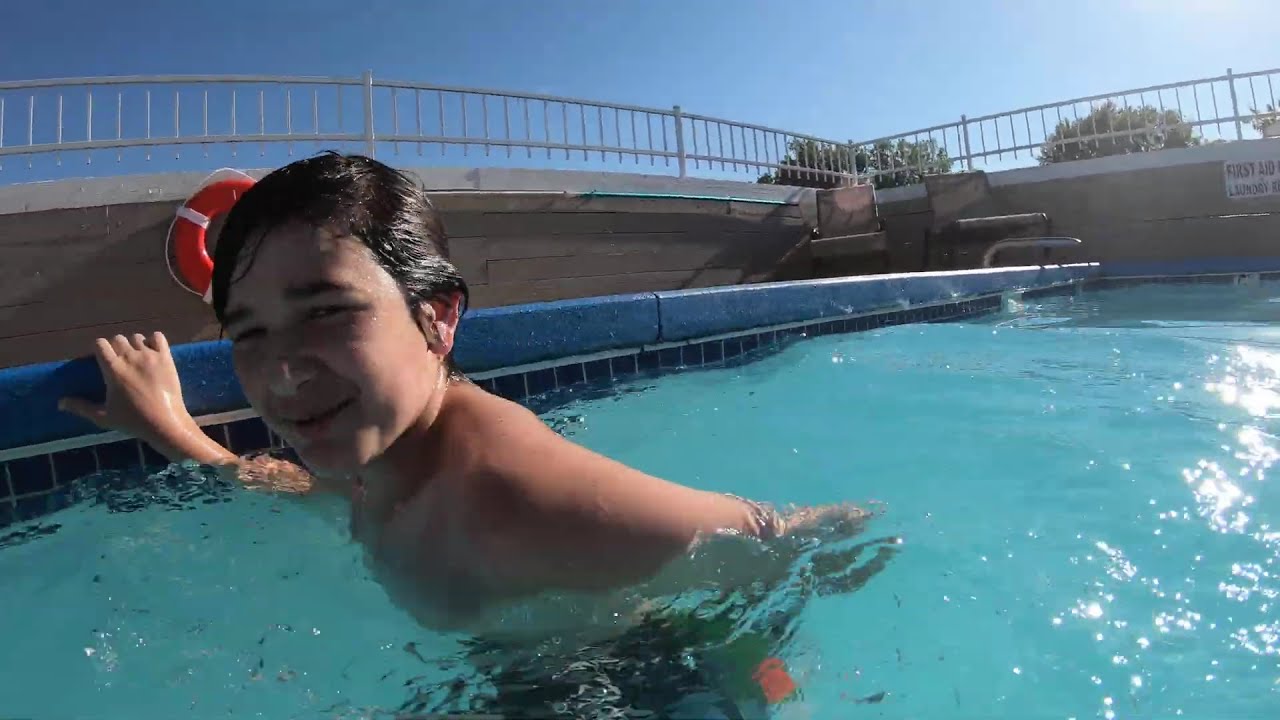This photograph captures a cheerful young boy, with wet, dark brown hair and olive skin, wading in a bright blue swimming pool. Positioned centrally, he looks directly into the camera, smiling, and holding on to the edge of the pool, suggesting he has just surfaced from underwater. Behind him, an orange and white life preserver is visibly mounted against a brown stone wall that surrounds the pool area. Above the life preserver, a white guardrail can be seen. To the right, near the corner of the pool, two little beach chairs are placed on the pavement. A sign labeled "First Aid" is also present on the far right, though the rest of the text is blurry. The pool's water is crystal clear, reflecting the bright sunlight. In the background, beyond the stone fence and chairs, lies a blue sky with some trees peeking over the top, capturing the essence of a sunny summer day.